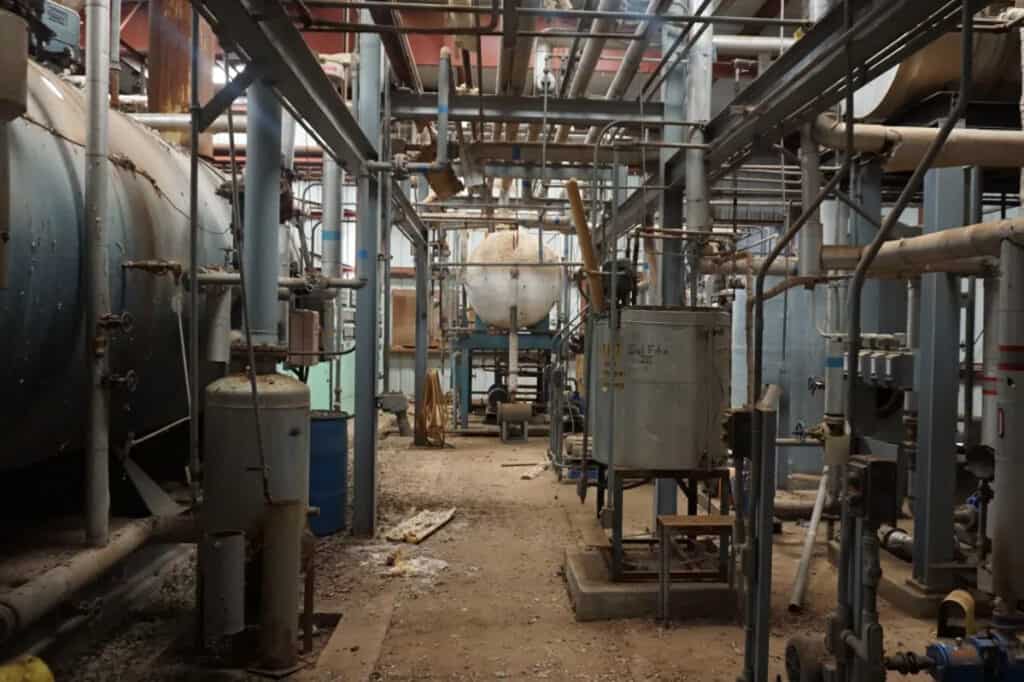The image depicts a well-lit industrial facility resembling a boiler room or factory. Sunlight streams through the windows, illuminating the expansive metal interior filled with intricate scaffolding and a maze of piping. Dominating the left side is a large black cylindrical tank with a complex pipe system that includes faucets and a T-joint leading to another pipe. Adjacent to it is a smaller silver cylinder connected by a vent pipe extending to the ceiling. In the middle right of the room sits a white cylindrical tank elevated on a metal platform, surrounded by blue barrels. The structure of the room includes horizontal metal bars on the ceiling and visible dirt on the factory floor, suggesting it's not in pristine condition. Additionally, a blue engine-like device is present on the far right. The facility appears devoid of people and seemingly inactive, adding a somewhat eerie feel despite the bright lighting.